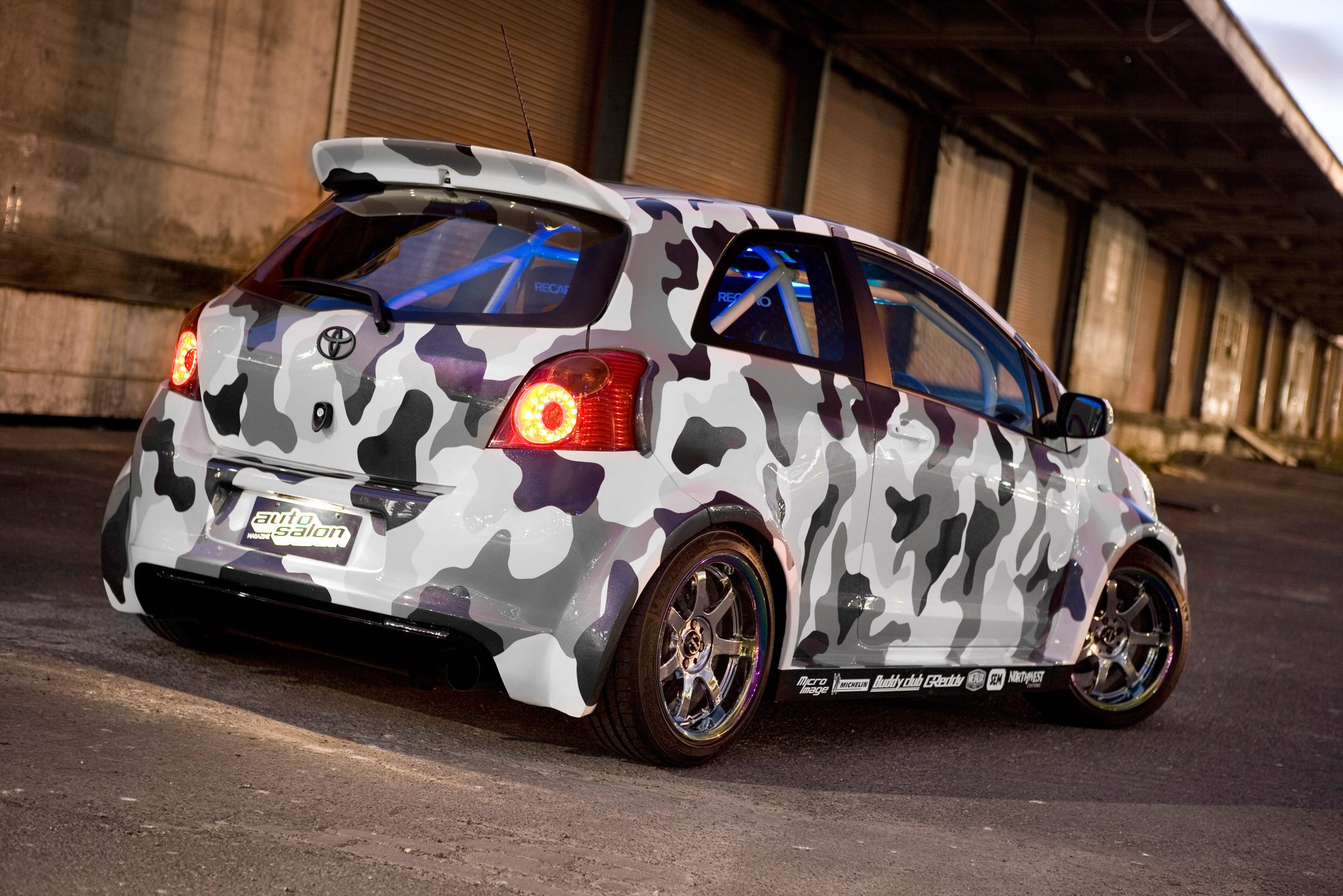This is a color photograph of a custom-painted Toyota hatchback, shown from the back at a diagonal angle, revealing both the rear and the right side of the vehicle. The car features a distinctive black, white, and gray camouflage pattern and sits low to the ground, indicative of modifications for racing. The rear brake lights are illuminated in red-orange, suggesting the brake is engaged. The vehicle's rims are metal with a sparkling chrome finish and exhibit luminescent purple and blue hues. Inside, the car is outfitted with a racing safety cage and has been modified to have only two seats, further emphasizing its racing capabilities. The black license plate reads "Auto Salon," likely indicating the garage responsible for these customizations. The background shows a large, possibly abandoned warehouse with corrugated iron shutter doors, situated on a tarmac surface. The scene is lit in dim, evening or morning light, with a small triangle of sky visible in the upper right corner, adding to the somewhat gloomy atmosphere.